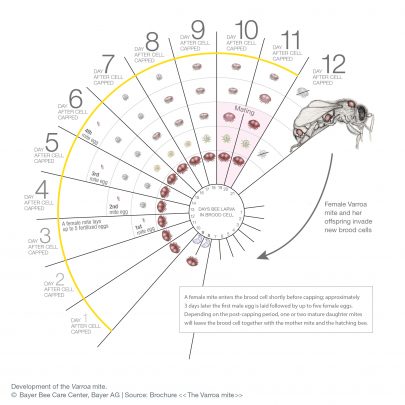The image is a detailed circular chart, resembling a semi-circle or half-clock, numerically marked from 1 at the bottom left to 12 at the top right, depicting the growth or progression of an insect, possibly a female Phagmos mite and her offspring. The semi-circle design features various colored sections with black lines delineating segments, and within these segments, there are red and gray dots potentially representing different stages or larva of the insect at each corresponding number.

At the end of this sequence at number 12, there is a fully developed insect, which appears to be fly-like with three distinct brown circles, large wings, and prominent black eyes. The color scheme includes black, white, red, yellow, gray, and brown, enhancing the details of the chart. A notable feature is the letter 'B' that stands out, hanging from one of the lines, and the chart itself is lined with black and yellow on its outer edge. Despite the intricate text and design elements, much of the writing within the chart is very small and hard to discern.